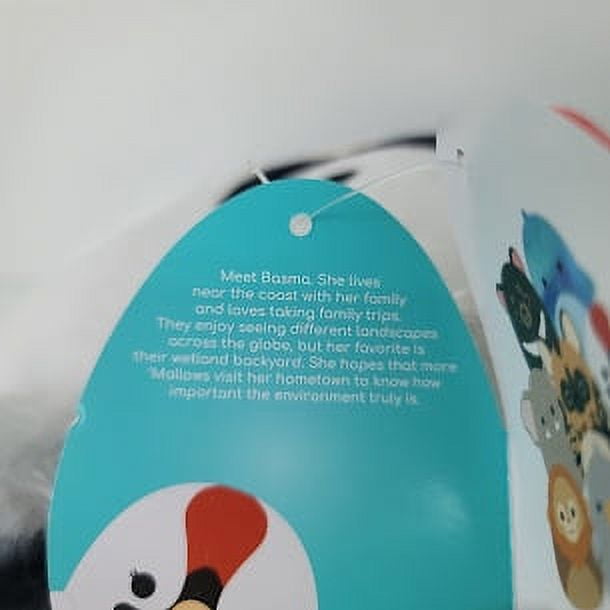The image shows a close-up of a blue tag attached to a child's toy, possibly a stuffed animal or Squishmallow, via a clear plastic tie. The text on the tag introduces a character named Basma, who lives near the coast with her family and enjoys taking family trips to explore different landscapes, with a particular fondness for their wetland backyard. Basma hopes more Squishmallows will visit her hometown to understand the importance of her environment. Despite the text's blurry appearance, you can make out these details. The bottom of the tag features a white animal with what looks like a rooster head, while the other side displays a collection of Squishmallows in a pyramid formation, including animals like a baby lion, elephant, bear, blue-haired bird, and a black bear. The tag's background is predominantly white with hints of red and black.